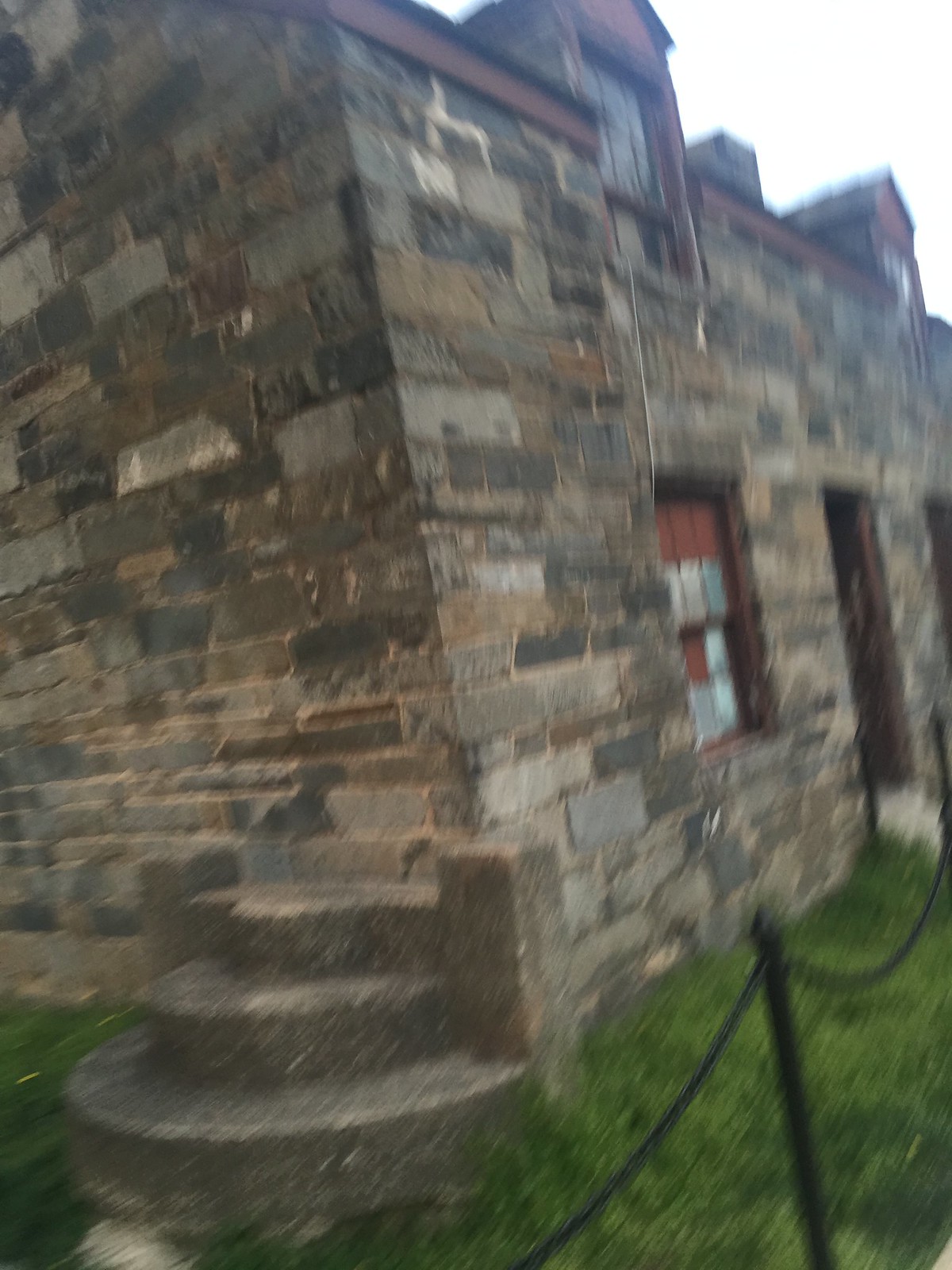This image showcases a somewhat blurry photograph of an outdoor structure, resembling an old castle. The first noticeable feature is a black, chain-link fence supported by poles, indicating a restricted area. The main building, viewed from its corner, is a two-story edifice constructed from a mix of gray, brown, and beige bricks, giving it a rustic, aged appearance.

The clearly visible side of the building includes three steps leading up to a wall with no entrance, emphasizing the corner perspective. To the right of this corner, there's a door serving as the main entrance. Adjacent to this door, a window is visible, notably sealed with dark and light materials. The top portion of this window is slightly open, revealing a light-colored segment covering the upper three-quarters.

The structure, with its medieval-like architecture, is surrounded by a patch of lush green grass, enhancing its historical ambiance.